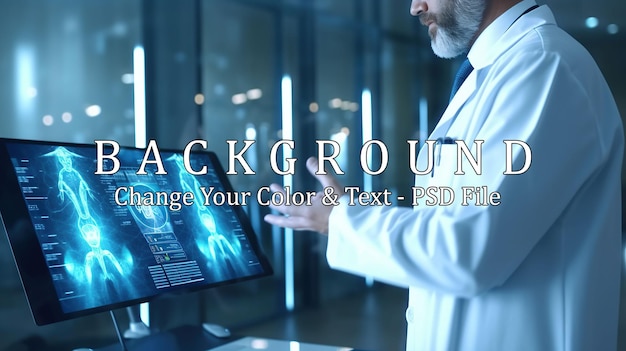The image depicts a close-up of an elderly man with a graying beard and mustache, dressed in a white lab coat over a white collared shirt and a light blue tie. Positioned on the right side of the frame, he's gazing to the left, revealing the side of his body and partially obscuring the view of his face beneath the nose. His lab coat's left pocket is filled with writing utensils. Behind him, the background text reads "change your color and text - PSD file."

On the left side of the image, there's a sleek, possibly touchscreen all-in-one computer situated on a countertop. The monitor displays a multi-section screen featuring an array of light blue images that resemble an exoskeleton or x-ray-like futuristic design, evoking thoughts of advanced technology or holograms. The man appears to be gesturing toward the monitor, which gives a sense of interaction, almost as if he’s engaged in a sophisticated task or explaining something. The overall scene is imbued with a blue hue, contributing to a technological and lab-like atmosphere, with a backdrop that includes glass and metal dividers suggestive of a modern office environment.